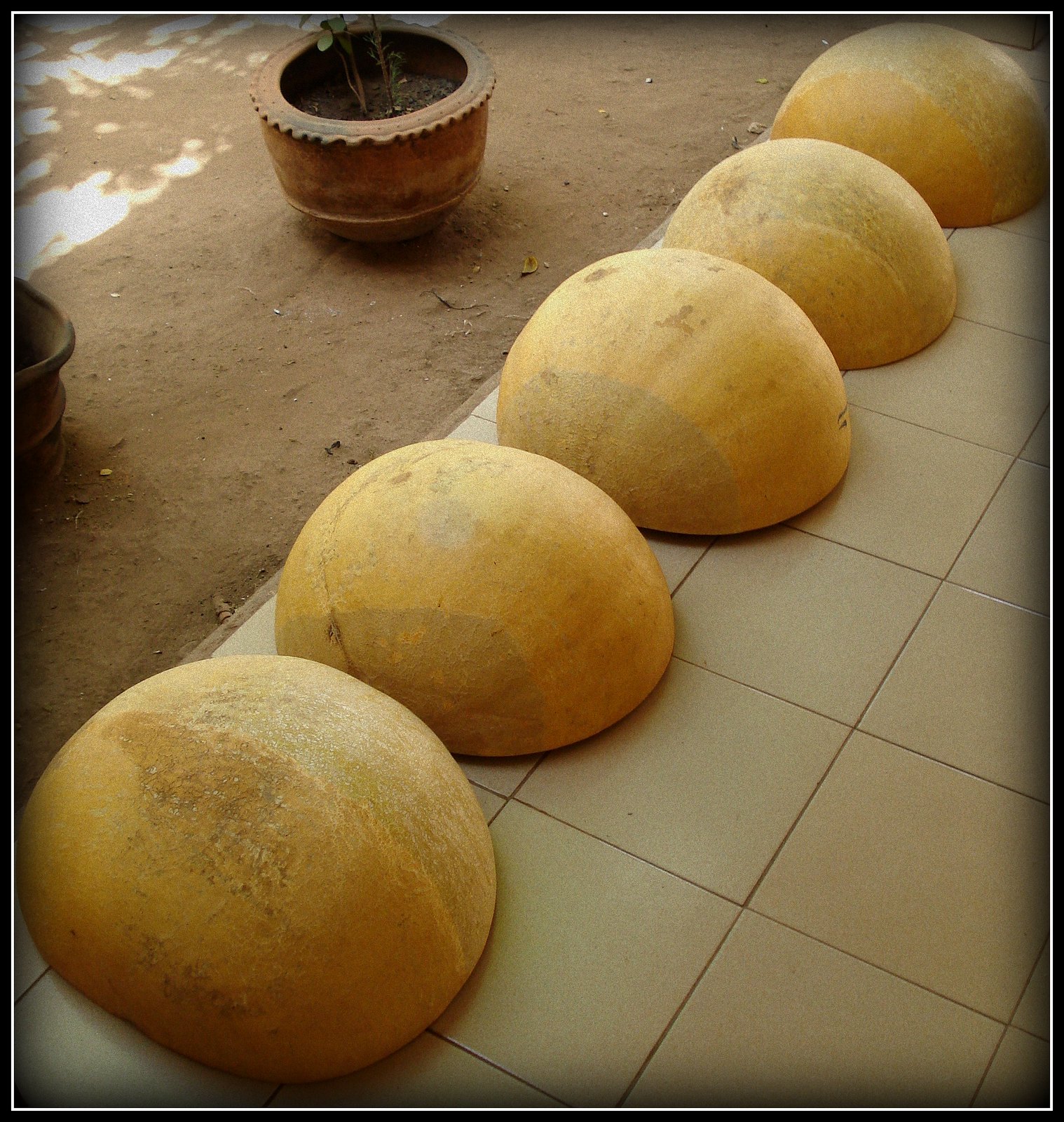The photograph captures five large, semi-circular objects resting flat side down on a white tiled surface, which resembles kitchen tile. These objects are intriguing because their appearance blurs the line between being pale yellow melons, flat stones, or possibly shells, each with some grayish circular markings and subtle veining. The upper left corner of the image shows a brown, scalloped-edged planter containing soil and a plant, and there is visible dirt adjacent to the tiles, creating an interesting juxtaposition of natural and manufactured elements.